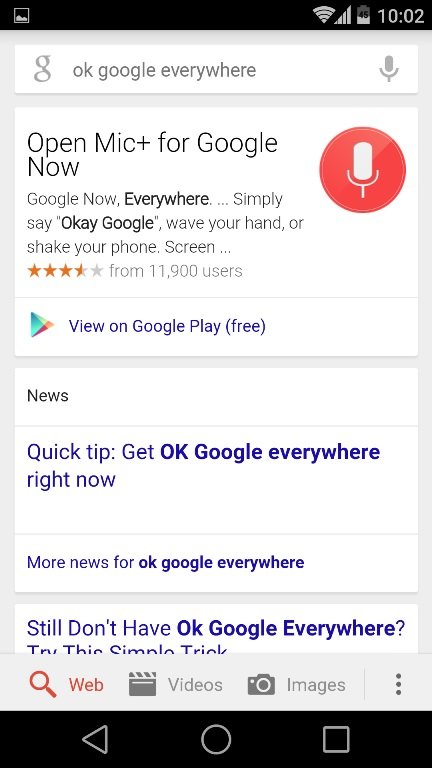This image is a screenshot, presumably taken from a cell phone. At the top, there is a black header featuring an image icon on the left, and Wi-Fi, full reception, half battery, and the time (10:02) icons on the right. Below the header, there is an "Ok Google" search bar. The screen prominently displays a white rectangle with black text reading "Open Mic+ for Google Now." Dominating the center is a large red circle with a microphone icon. The text states, "Google Now everywhere: simply say 'Ok Google,' wave your hand, or shake your phone screen." The app has garnered an average rating of three and a half stars from 11,900 users. Additionally, a news blurb at the bottom provides a quick tip: "Get 'Ok Google' everywhere right now."